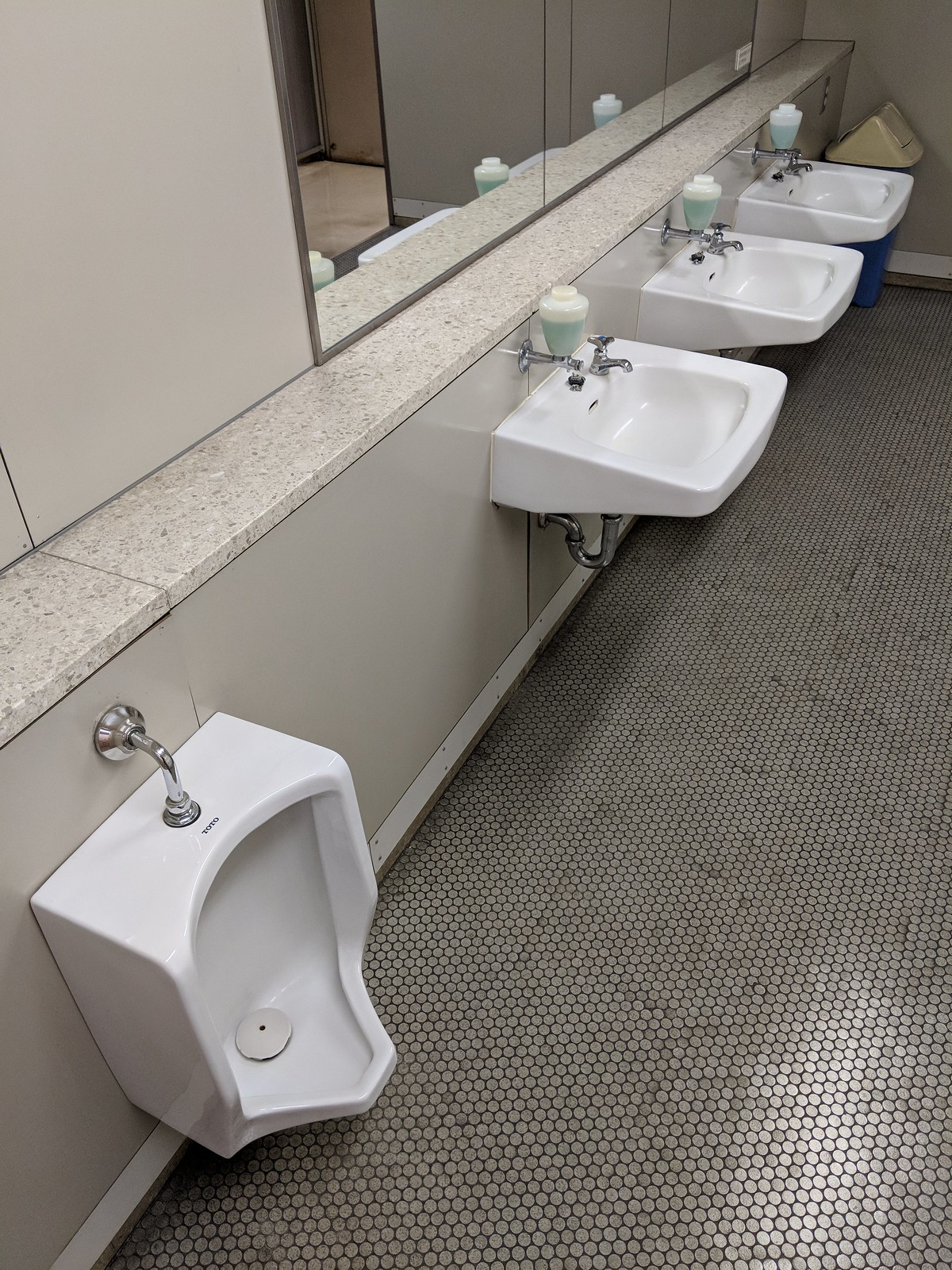This image depicts a children's bathroom, likely situated in a school. The left side of the image shows a white urinal, positioned low to the ground with silver piping and containing a urinal cake, indicative of a child-friendly design. The floors are covered in small, grayish penny tiles, which appear somewhat dirty with blackened grout. Beige walls frame the room, with gray tiles running along the base and meeting up with a large mirror that dominates the central portion of the wall.

Below the mirror are three white sinks, each mounted directly to the wall, with visible silver plumbing underneath. The sinks feature silver faucets, likely designed to conserve water by automatically shutting off. Topping these sinks are lime-green soap dispensers with white caps, adding a pop of color to the otherwise muted palette.

Further to the right, partially seen in the image, is a blue and white wastebasket containing a brown box. This functional layout ensures cleanliness and order, accommodating the practical needs of a space frequented by children.